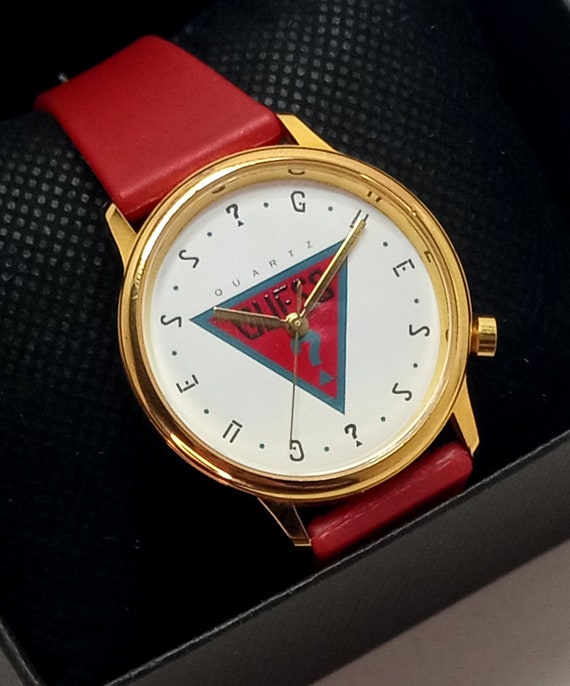This detailed color photograph captures a luxury watch that exudes elegance and sophistication. The watch, branded by Guess, features a striking gold-rimmed face adorned with gold hands, including a second hand. Unique symbols replace the traditional numbers, with prominent question marks and the letters G-U-E-S-S around the dial. The face of the watch is white, highlighted by an upside-down red triangle outlined in blue, displaying the Guess logo in black, with "Quartz" written above it. Complementing its refined face, the watch has a vibrant red leather strap. Presented in a sleek black gift box with a ridged texture, the watch rests gracefully on a black pillow, enhancing its luxurious appearance. Professionally lit against a white background, the photograph eloquently captures the watch's 90s-inspired design, emphasizing its classy and expensive aesthetic.